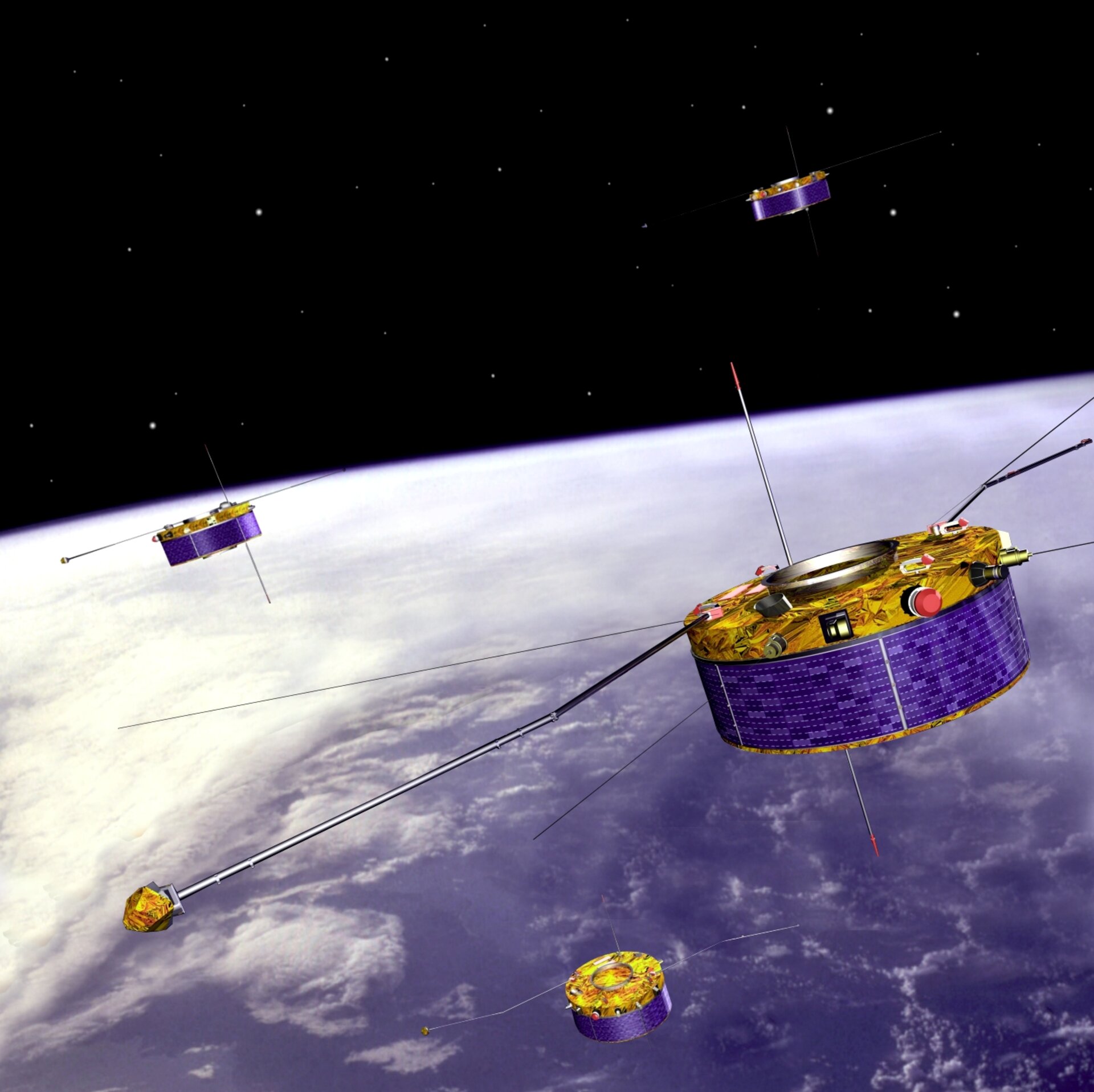The image is a detailed, computer-generated scene of space, featuring four identical satellites in orbit above Earth. Earth occupies approximately the lower two-thirds of the frame, with a pale blue surface mottled by white clouds, juxtaposed against the black backdrop of space speckled with stars. Each satellite is a relatively flat cylinder, about a third or a fourth as tall as it is wide. They exhibit a distinct purple rim adorned with a gradient of purple box-like designs, and their tops are gold and silver with intricate multicolored patterns, featuring red circles and small black squares. Teeming with detail, each satellite has metal rods and antennas extending horizontally from its top. One satellite is prominently in the foreground on the right-hand side, while the other three, smaller due to perspective, hover directly above the visible part of the planet. The organized placement and identical appearance of these satellites against the serene expanse of Earth and space create a strikingly detailed and captivating scene.